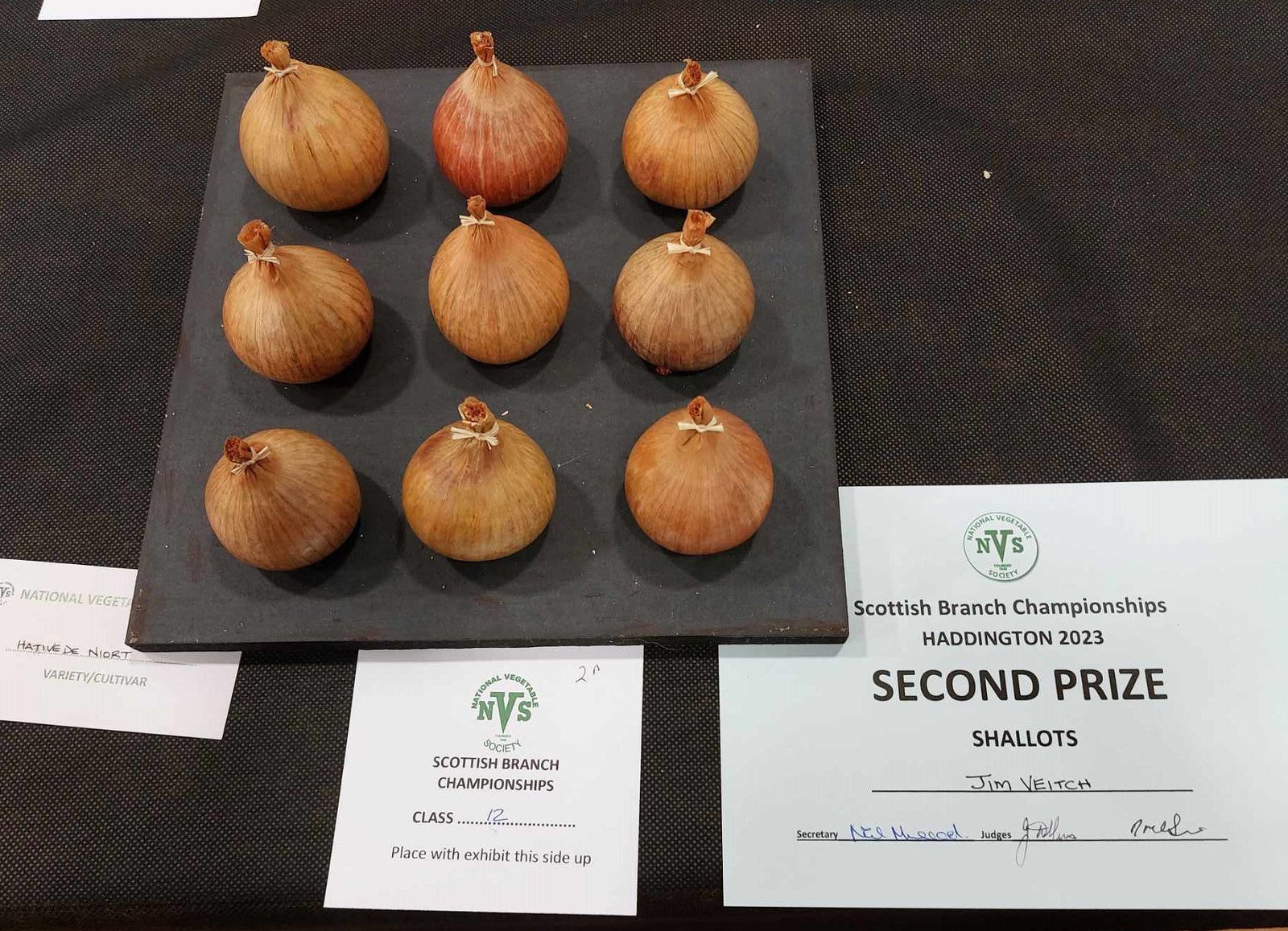This rectangular photograph captures a winning display from the National Vegetable Society's Scottish Branch Championships. On a square black platform draped with a dark cloth, we see nine meticulously arranged shallots positioned in a three-by-three grid on a dark metal platter. Below the platter, three placards provide details about the entry. The largest placard on the right reads "Scottish Branch Championships Haddington 2023, Second Prize, Shallots," along with the name of the winner, Jim Veitch, and signatures from the judges and secretary. The middle placard indicates "National Vegetable Society Scottish Branch Championships Class 12" and instructs to "Place this with exhibit this side up." To the left, a partially concealed placard likely details the variety and cultivar of the shallots displayed. This precise arrangement and detailed labeling highlight the care and effort put into this prize-winning exhibit.